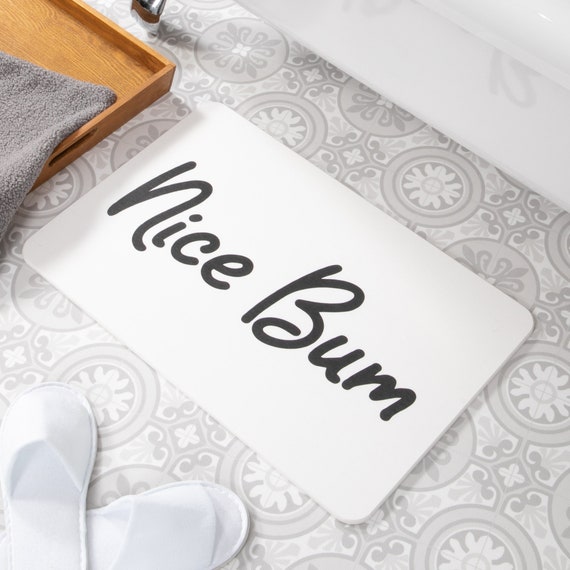This image is a detailed, close-up, indoor color photograph of a bath mat on a tiled bathroom floor. The bath mat is white and appears to be made of memory foam. In neat, cursive-like black lettering, it reads "nice bum." The floor tiles are in shades of gray and white, featuring a Spanish-style, floral pattern. In the lower left corner, there is a pair of white slip-on slippers. In the upper right, part of a bathtub is visible, confirming the bathroom setting. A wooden tray with a blue towel is positioned on the left side of the mat, adding context to the scene. The overall color palette of the image is predominantly white and off-white, with natural tones from the wooden tray and subtle blue accents from the towel.